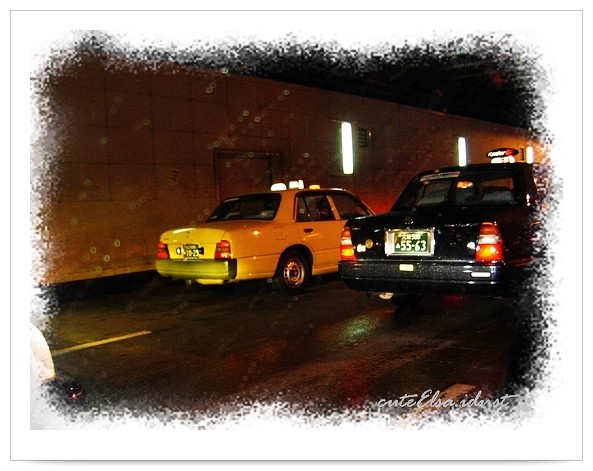The image depicts a nighttime scene of two taxis driving through what appears to be a tunnel during a rainstorm, as indicated by the wet pavement and visible raindrops. One taxi is a traditional yellow cab, complete with typical taxi markings, a rooftop sign, and a license plate. The other taxi is a black, boxy vehicle, possibly belonging to a private cab company, which also sports a rooftop sign with white writing and a red image, and a distinctive short license plate that reads "55-63." The road features a dashed white line and a large concrete divider with rectangular white lights hanging from it. The tunnel wall on the right side of the image shows two or three small windows. The photograph has an artistic quality, with a smeared white border added through Photoshop, evoking a blend of black and white splotches around the edges. The entire composition is framed within a square shape, adding to its artistic presentation.